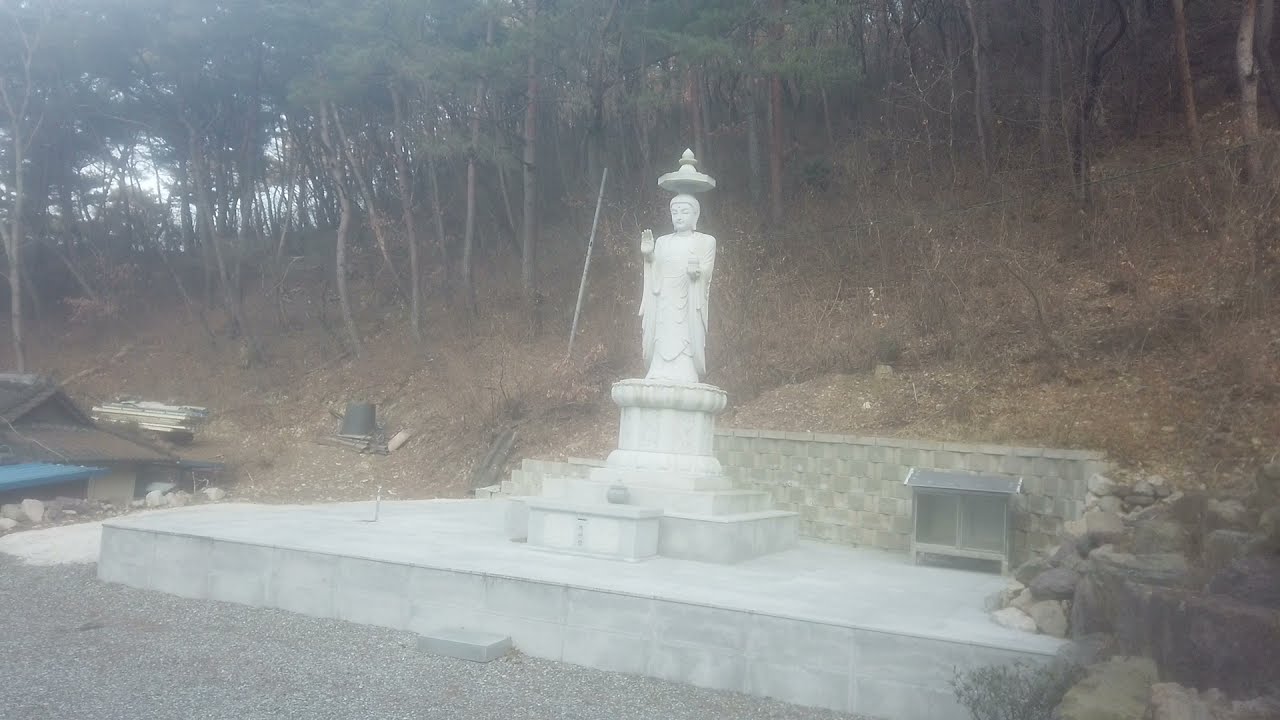The image depicts an outdoor scene centered around a white statue of a person, possibly of South Asian or Indian origin, given the dot on the forehead. The statue stands on a concrete pedestal atop a larger cement block, which is set against a background of a wooded hillside filled with trees. The trees vary in thickness, with some showing skinny trunks, and the sky with some clouds can be glimpsed through the branches, giving the scene a slightly hazy appearance. The figure in the statue holds their right palm up and carries a box or trinket in their left hand. Above their head, there is a circular base with a pointed top, which might be a fountain or another decorative element. Surrounding the statue are various construction materials and debris; to the left, there are plywood boards, a bucket, and what looks like a discarded steel grate, while to the right, there are some bricks. The ground around the pedestal is mainly covered in stone or gravel, contributing to the overall rugged and unfinished look of the area.